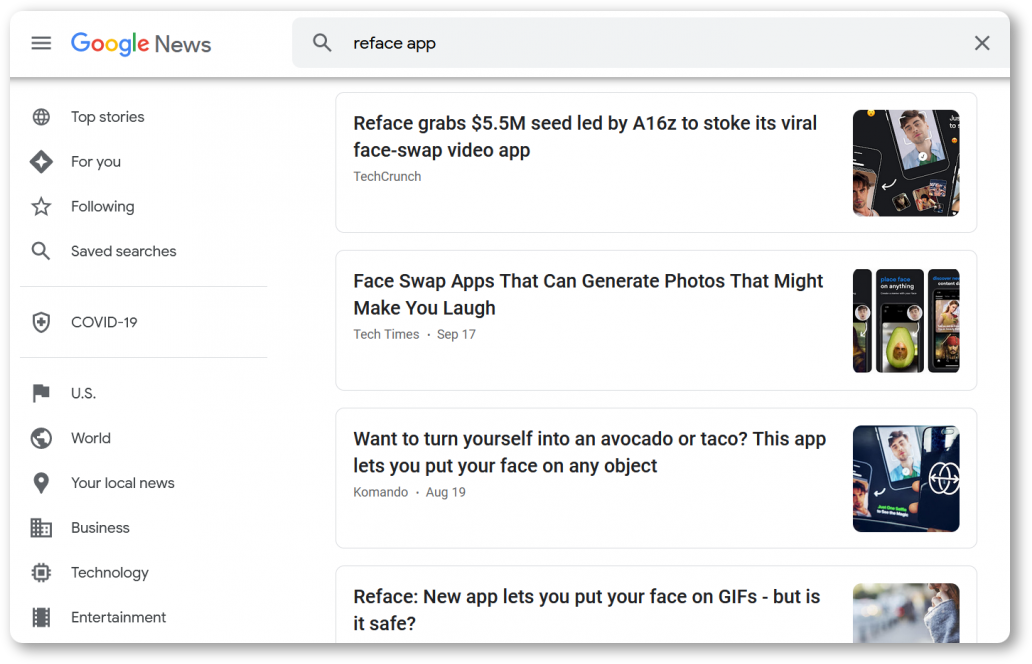This horizontal screenshot captures a Google News page, focusing on the "Reface App." In the top-left corner, the familiar multicolored Google logo is paired with a gray-font "News," adjacent to a menu icon formed of three horizontal bars. Directly to the right is a search bar displaying the query "Reface App" in black font.

On the left sidebar, a series of icons accompanies various categories, listed from top to bottom: Top Stories, For You, Following, Saved Searches, COVID-19, U.S., World, Your Local News, Business, Technology, and Entertainment.

The main content on the right features a series of article snippets. Each headline is presented in bold black font within a horizontal white rectangle, flanked by an image on the right. The first article, titled "Reface grabs $5.5M seed led by A16Z; it's dope, it's viral, face-swap video app" from TechCrunch, is accompanied by an image showing cell phones displaying various faces. The second article, "Face-swap apps that can generate photos that might make you laugh," comes from Tech Times, dated September 17th, with the accompanying image depicting three cell phones. The third article, "Wanna turn yourself into an avocado or taco? This app lets you put your face on any object," is from Commando, dated August 19th. The last article on the list is titled "Reface, new app lets you put your face on GIFs, but is it safe?" and lacks further details.

The layout and design are efficient, offering a seamless reading experience with visual aids that enhance each article snippet.